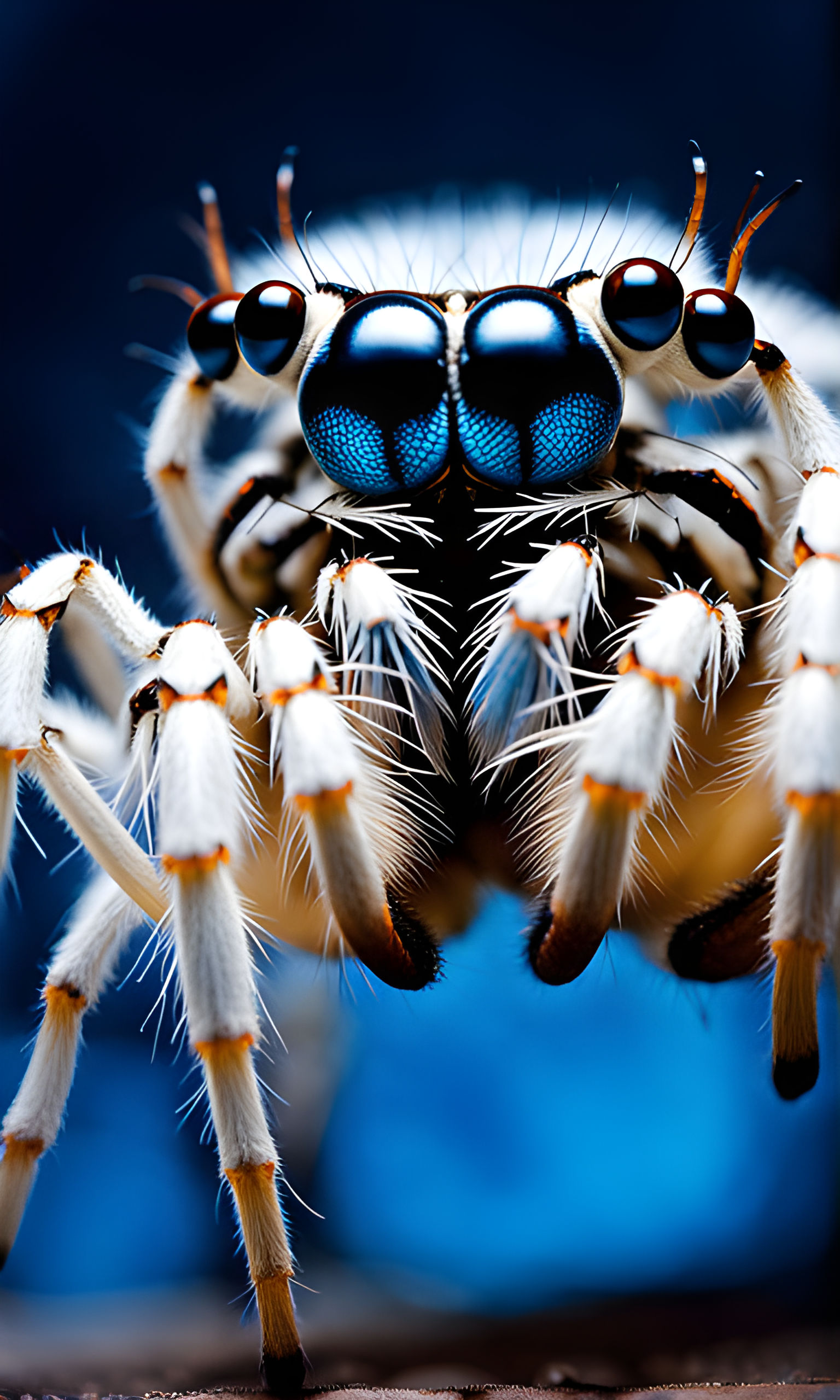This is an extremely detailed, up-close photograph of what appears to be a white spider with orange segments on its legs. The spider has six eyes, which are prominently displayed in the image: two large ones in the center flanked by two smaller eyes on either side, featuring a mesmerizing combination of deep blue and black. Its fur-like hairs are meticulously clear, and several antennae protrude from its head, totaling four or five. The composition makes the viewer feel as though they're gazing directly into its eyes, with the perspective capturing a first-person view. The spider's mouth, flanked by two fangs, is visible and adds to the intimidating appearance of the creature. The background enhances the eeriness with a bluish-black hue at the top and a blurred lighter blue towards the bottom, giving a sense of nocturnal mystery. The spider seems to be in motion, with some legs in the air, and positioned as if standing on an indistinct surface. This vivid image, whether a photograph or AI-generated, conjures a very lifelike and terrifying appearance.